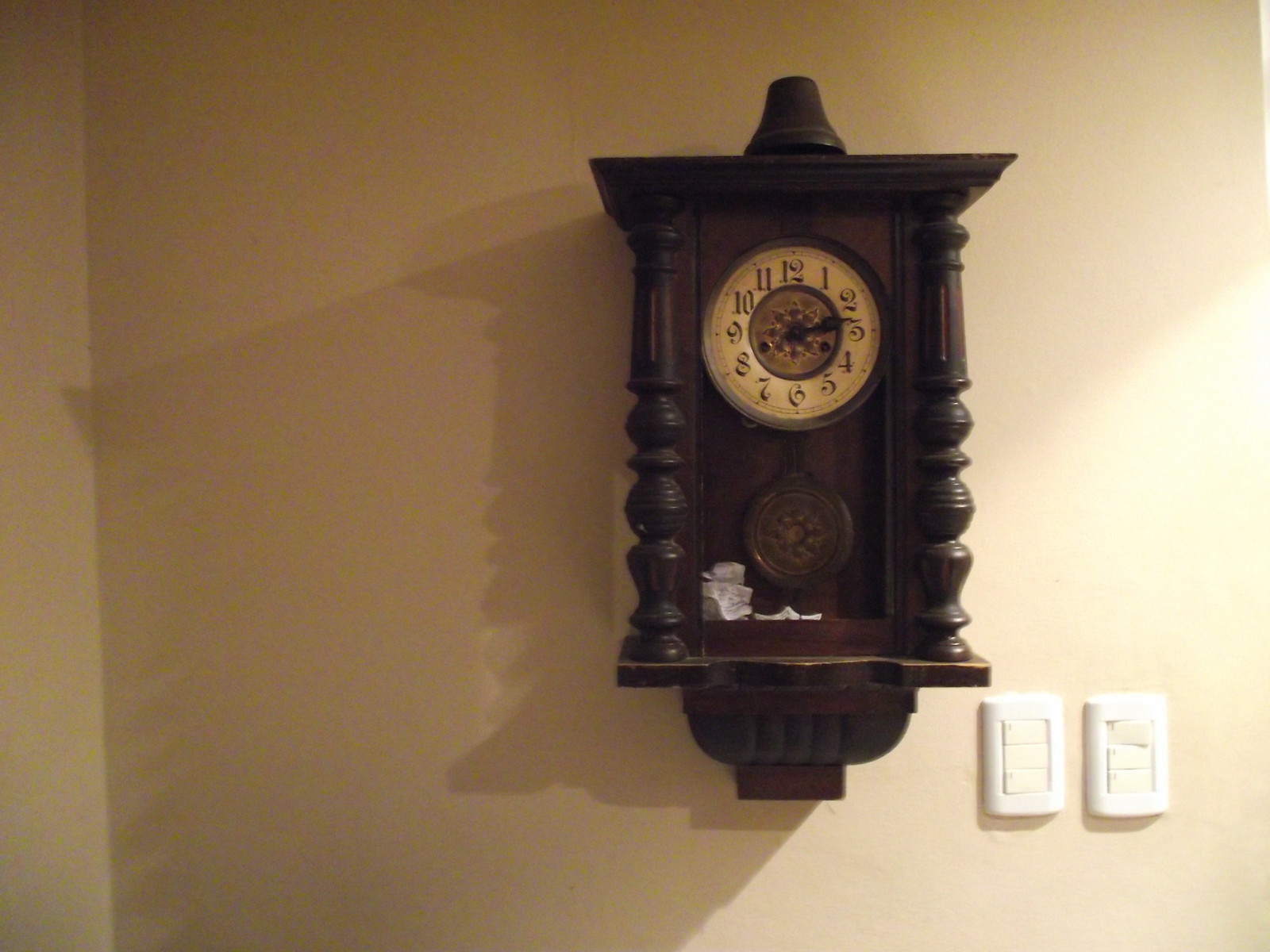This photograph captures an antique-style pendulum wall clock that resembles a miniature curio cabinet. The clock, housed in a rectangular, cherry-colored wooden case with ornate, bulbous columns on either side and a conical top, is set against a pale yellow or beige wall. Its face is light-colored, featuring black, slightly scrolling numbers from 1 to 12, with a star-like detail in the center. The clock shows approximately 2:13. Below the dial, there's a small wooden pendulum with a wide, possibly metal, disc at the bottom. Additionally, a bell is positioned underneath the clock face, with some type of paper or tissue within the wooden case. Slight shadows extend to the left of the clock, indicating a light source from the middle right of the image. To the bottom right of the clock, two light switches with three white horizontal buttons each are visible, adding to the details of the wall setting.